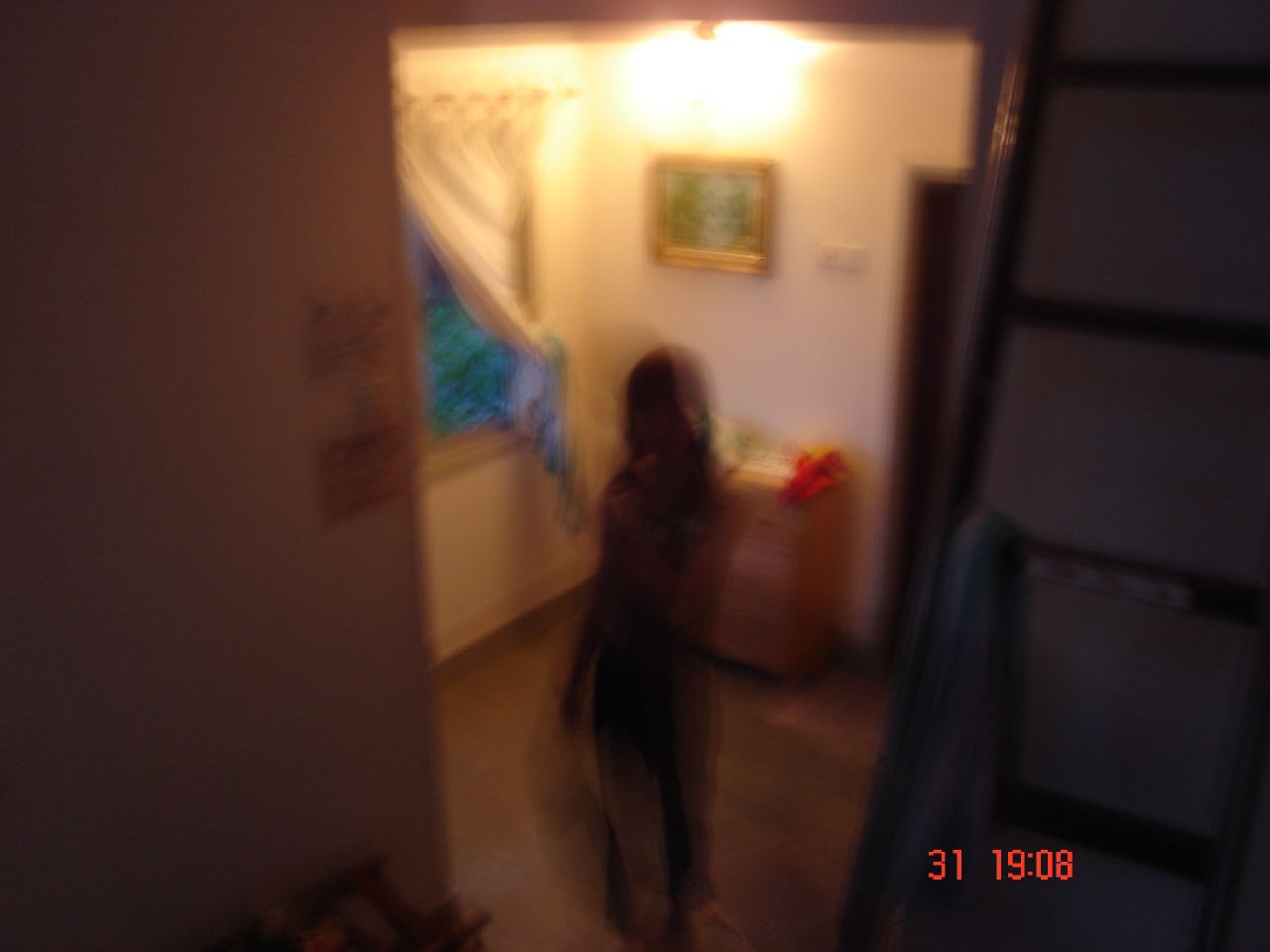The image captures a blurry and somewhat eerie scene that evokes the impression of a ghostly apparition. Predominantly, the blur creates a surreal effect, almost as if a young girl's spirit is faintly separating from her body. A soft light illuminates the middle of the room, casting shadows that add to the mysterious atmosphere. There appears to be a gentle breeze coming through a window, contributing to the movement captured in the photo. In the background, a painting hangs on the wall beside a small cabinet, but these details are obscured by the overall blur of the image. The intentional or unintentional camera movement has resulted in a composition that could easily deceive the viewer into believing it depicts a paranormal event.